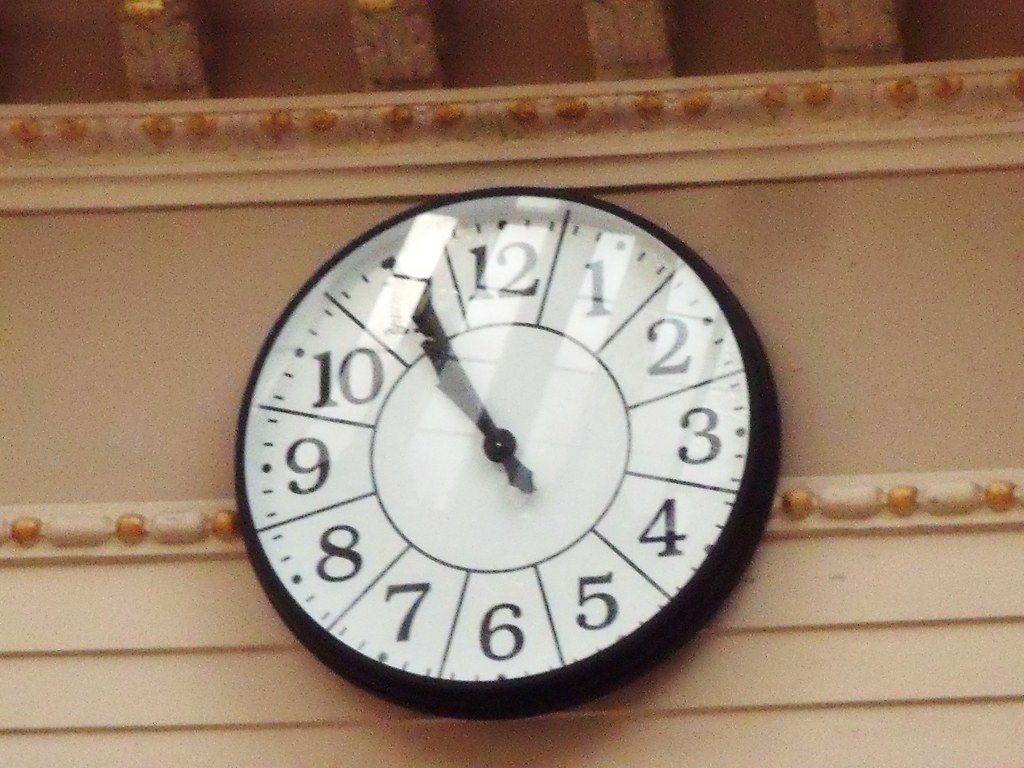The image depicts a wall painted in a cream or beige color with a horizontal ornamentation at the top and mid-section. This decoration consists of alternating gold oval beads and silver oblong beads. Below this decorative element, the wall features a lighter beige paneling or siding. Prominently displayed on the wall, between the upper and middle sections, is a clock. This clock has a white face, black numbers, and black hands, all housed within a black plastic border. The time displayed on the clock is approximately 10:50 to 10:53, and there is a slight glare on its surface.